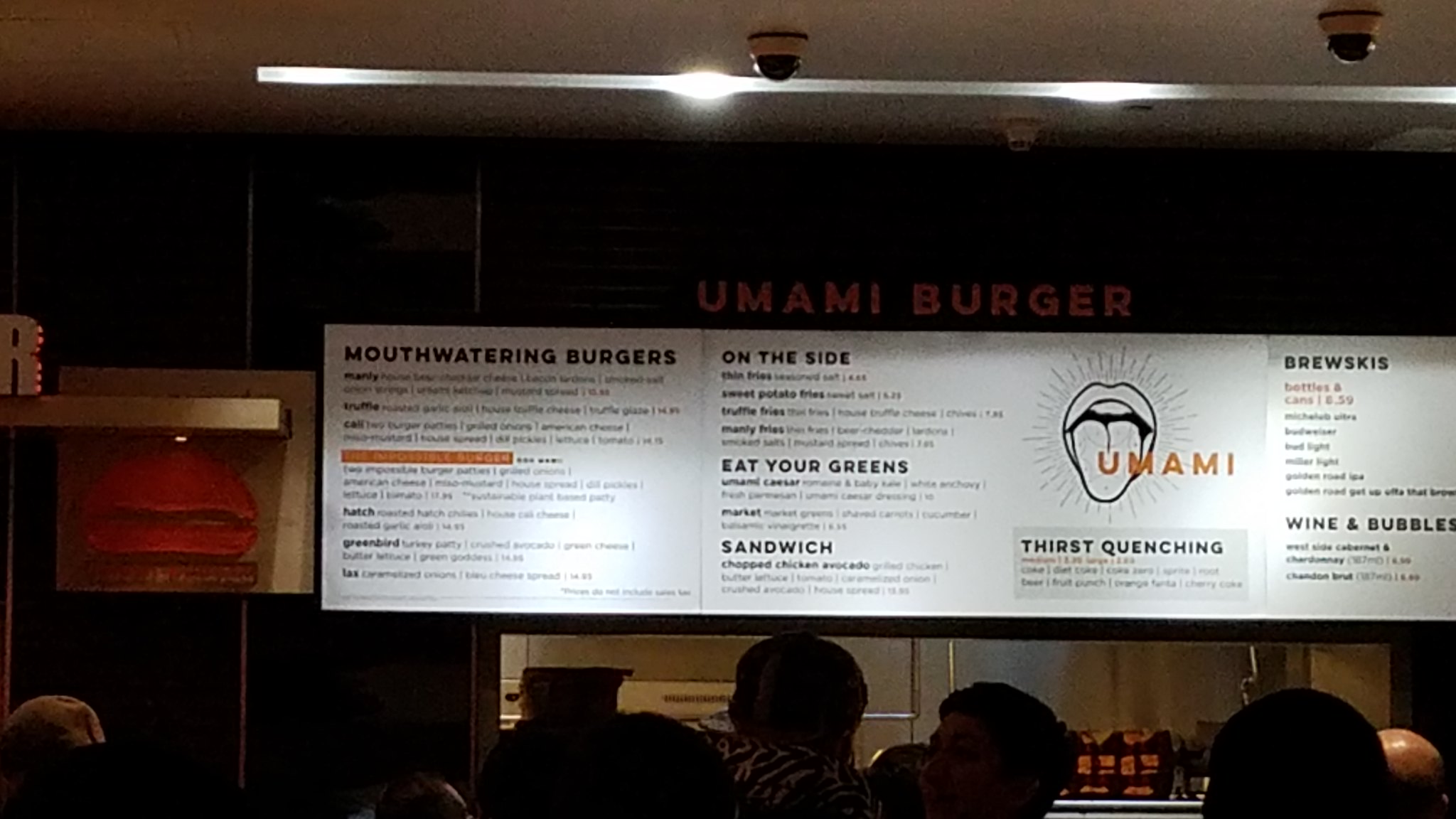In this dimly lit restaurant, a vibrant and illuminated menu board hangs prominently above the counter, casting a warm glow in the otherwise subdued ambiance. The ceiling is adorned with a bar of lights and a few security cameras, adding to the practical yet somewhat shadowy environment. Among the cropped heads and shoulders of waiting patrons, a few taller individuals stand out in the line, their features indistinct but detectable.

On the left side of the image, a framed picture of a burger decorates a dark-colored wall. A shelf below this artwork displays freestanding illuminated letters, the only discernible one being an 'R,' likely part of the word 'BURGER.' The back wall, painted in a dark hue, features a large double open window providing a glimpse into the bustling kitchen where culinary preparations are underway.

The menu board is composed of four white illuminated panels. The first panel proclaims "mouth-watering burgers" and lists various burger options, though they are too distant to read clearly. The second panel, labeled "on the side," details side dishes, followed by "eat your greens," presumably for salads, and a selection of sandwiches. The third panel showcases a whimsical illustration representing "umami," with a cartoonish open mouth and tongue radiating energetic rays, the word 'UMAMI' playfully integrated into the design. Underneath, it reads "thirst-quenching," hinting at beverage options. The fourth and final panel, titled "brewskis," lists the beers available, with "wine and bubbles" featured below.

Amidst this inviting scene, roughly half a dozen individuals wait in line. One young person, whose gender is indeterminable, has their head turned to the left. In the very right bottom corner, a bald-headed patron stands out, the overhead light reflecting off their scalp. The overall image captures a bustling yet cozy atmosphere focused around the enticing promise of delicious food and drink.